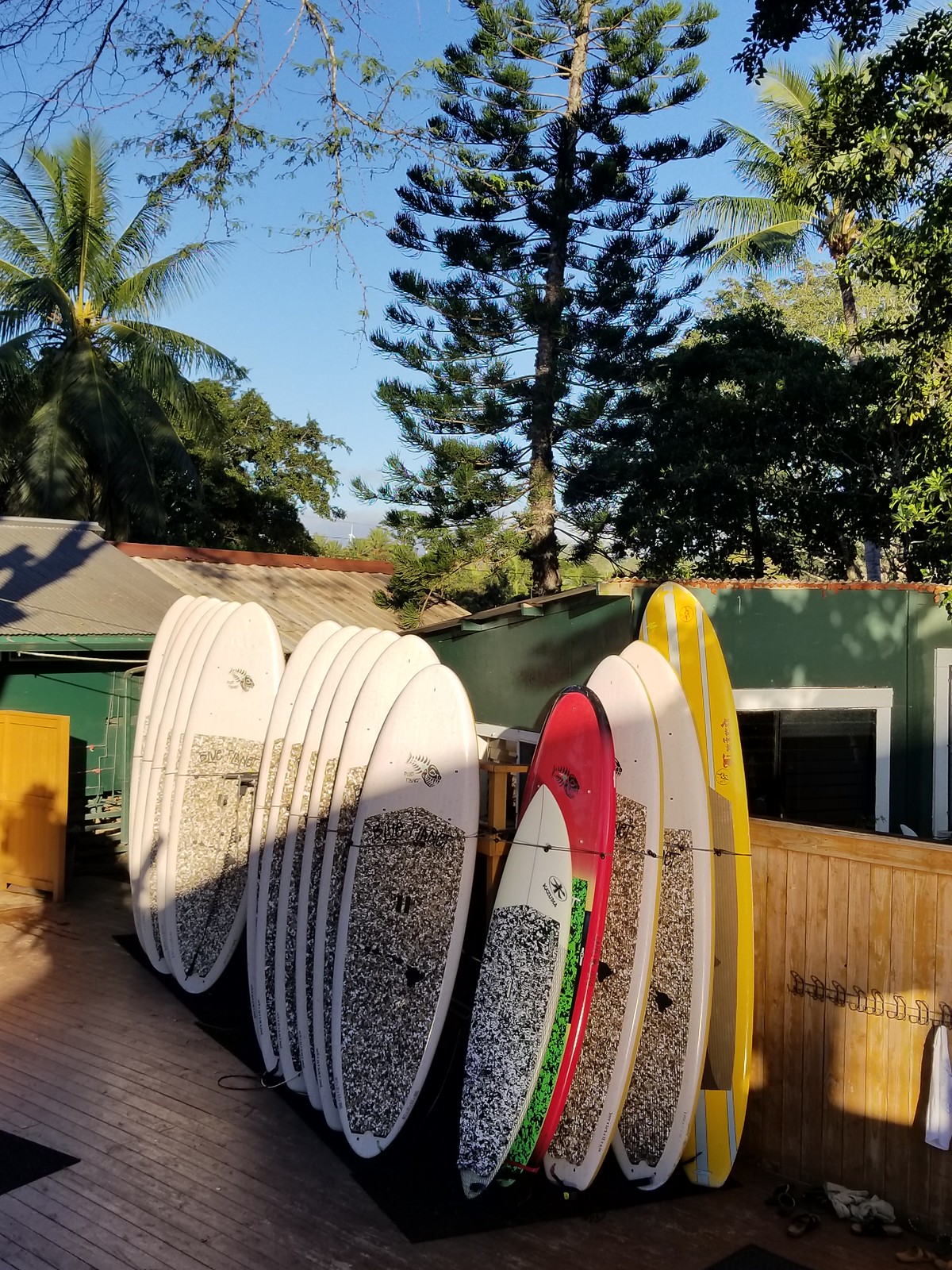In this photograph taken in a tropical location, a large collection of surfboards and paddle boards are neatly lined up against a light brown cedar fence with a top rail. The boards are arranged on a wooden deck that stretches from the bottom right to the left middle of the image. The majority of the boards are tall and white, featuring intricate black ink designs that resemble a bee-like pattern, although the details of these designs are not clearly visible due to the distance of the shot. There is a notable variety in the collection: one surfboard stands out in hot pink with a V-shaped design in the center flanked by pink and yellow backgrounds, and another board, the tallest of them all, is yellow adorned with white stripes and beige sections.

Beyond the fence, the scene includes green buildings with corrugated tin roofing and white trim around the doors and windows. One of these buildings features a yellow door. The vibrant backdrop is completed with an array of trees, including palm trees, deciduous trees with dark and light green leaves, and a pine tree. The trees cast long shadows over the buildings, boards, and deck, suggesting the photograph was taken later in the day under a beautiful blue sky that fades to a lighter shade towards the horizon.